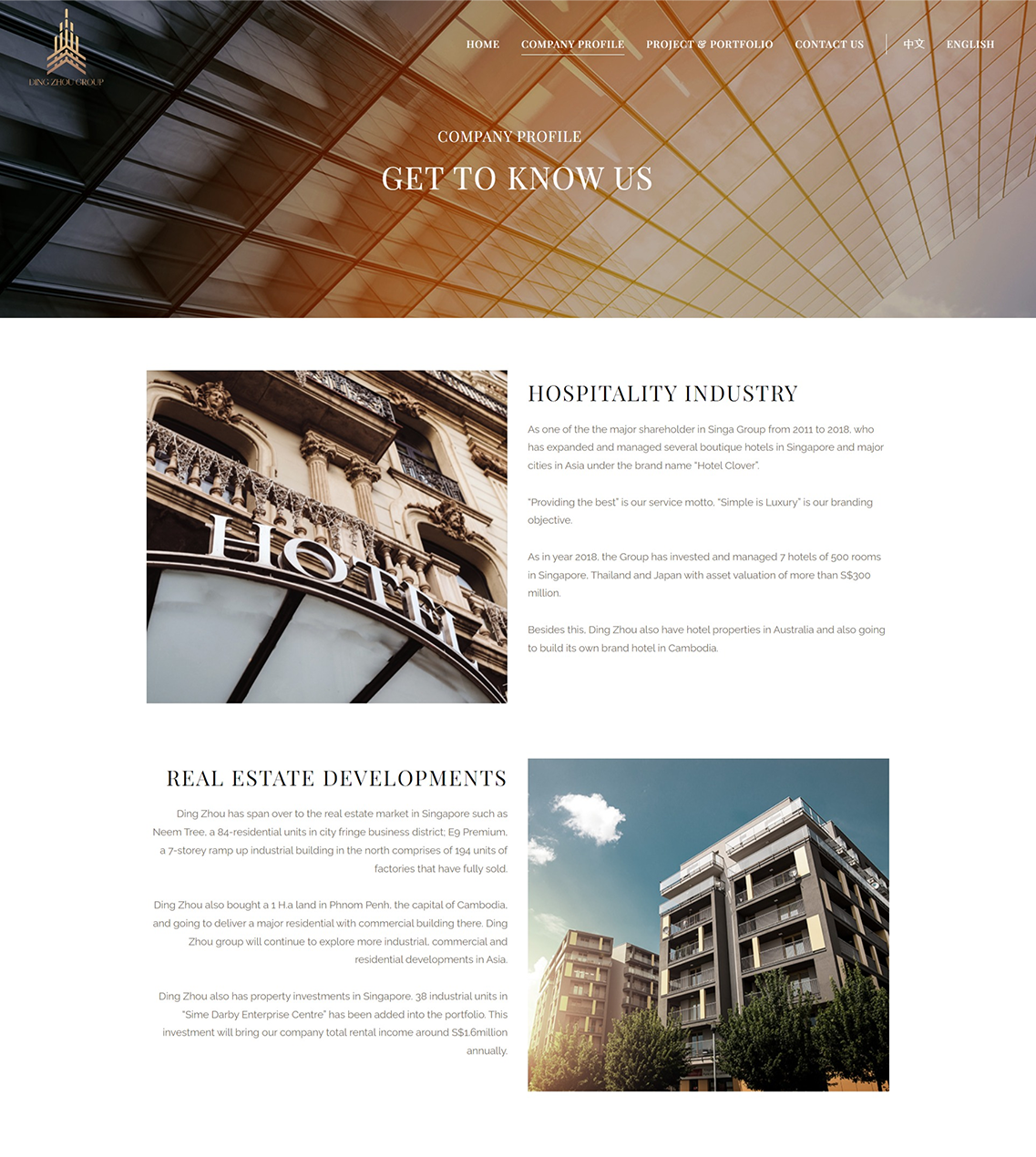In this image, we see the top left logo for Lion Zoo Group, also known as LingZoo Group. The prominent categories on this page include Home, Company Profile, Project and Portfolio, Contact Us, English, and an Asian language. The Company Profile section encourages visitors to "Get to Know Us" and highlights their expertise in the hospitality industry. As a major shareholder in Singa Group from 2011 to 2018, LingZoo Group has expanded and managed several boutique hotels in Singapore and major cities across Asia under the Hotel Clover brand. Their service motto is "Providing the best," and their branding objective is "Simple is luxury." By the year 2018, the group had invested in and managed seven hotels with a total of 500 rooms in Singapore, Thailand, and Japan, holding assets valued at over $300 million. Additionally, LingZoo Group has hotel properties in Australia and is planning to establish its own brand in Cambodia.